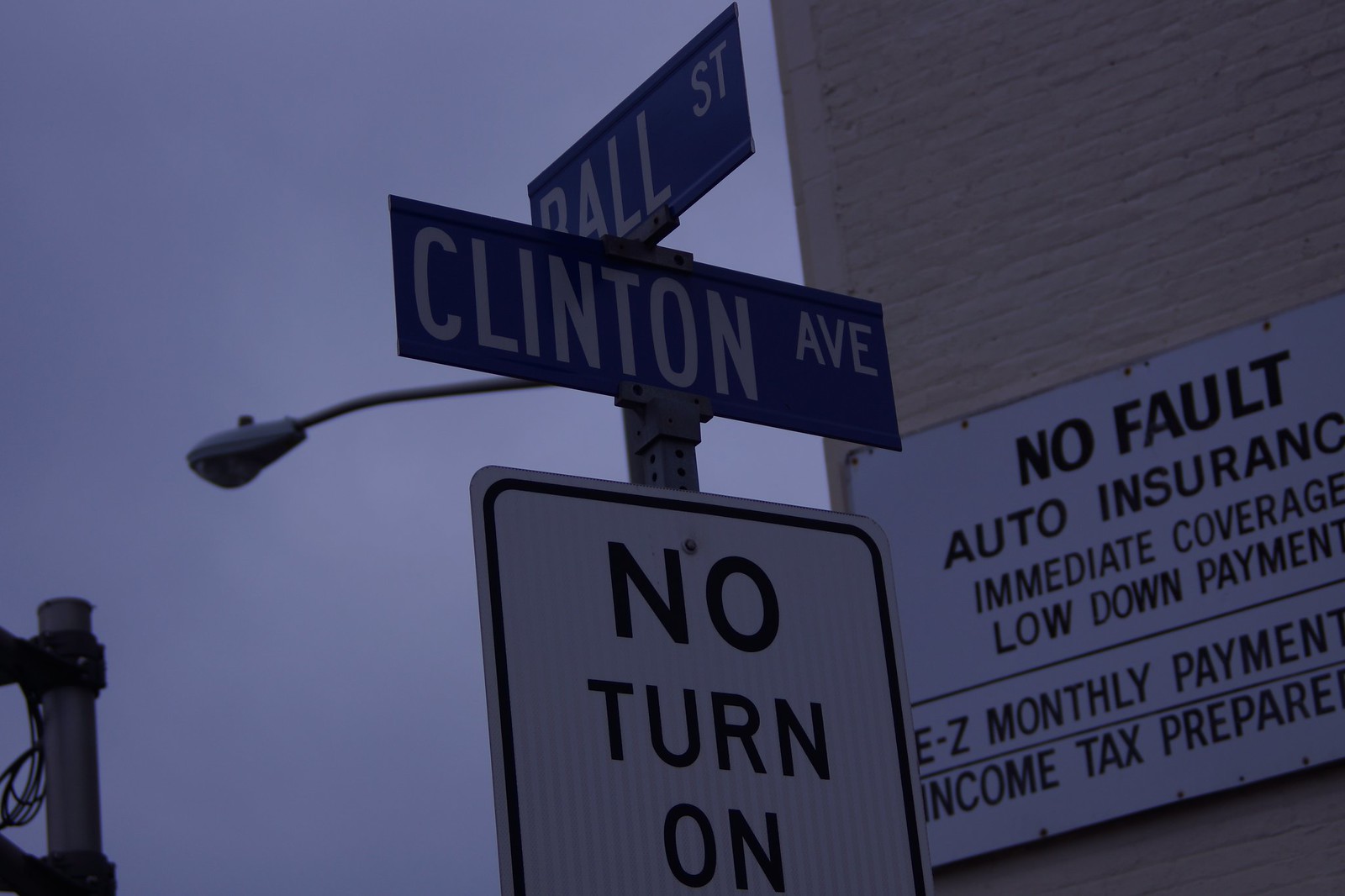In this image, we see a street corner under an overcast sky with a thick layer of clouds, suggesting an approaching evening. On the right side, a tall brick building painted in a pale cream color dominates the scene. Affixed to the building is a large white sign with red and black text advertising "No Fault Auto Insurance, Immediate Coverage, Low Down Payment." Below this, separated by a black line, are the words "E-Z Monthly Payments" and "Income Tax Prepared."

Central to the image is a metal pole with several signs. At the top are two blue street signs with white letters, indicating the intersection of Ball Street and Clinton Avenue. Below these, a rectangular white traffic sign with a black border reads "No Turn On," though the rest of the message is not visible.

To the left of this pole, there's a tall street light, adorned with black hooks around its top, which hasn't been illuminated yet. The overall scene is tinged with the muted light of a late or dim time of day, adding a somber tone to the image.